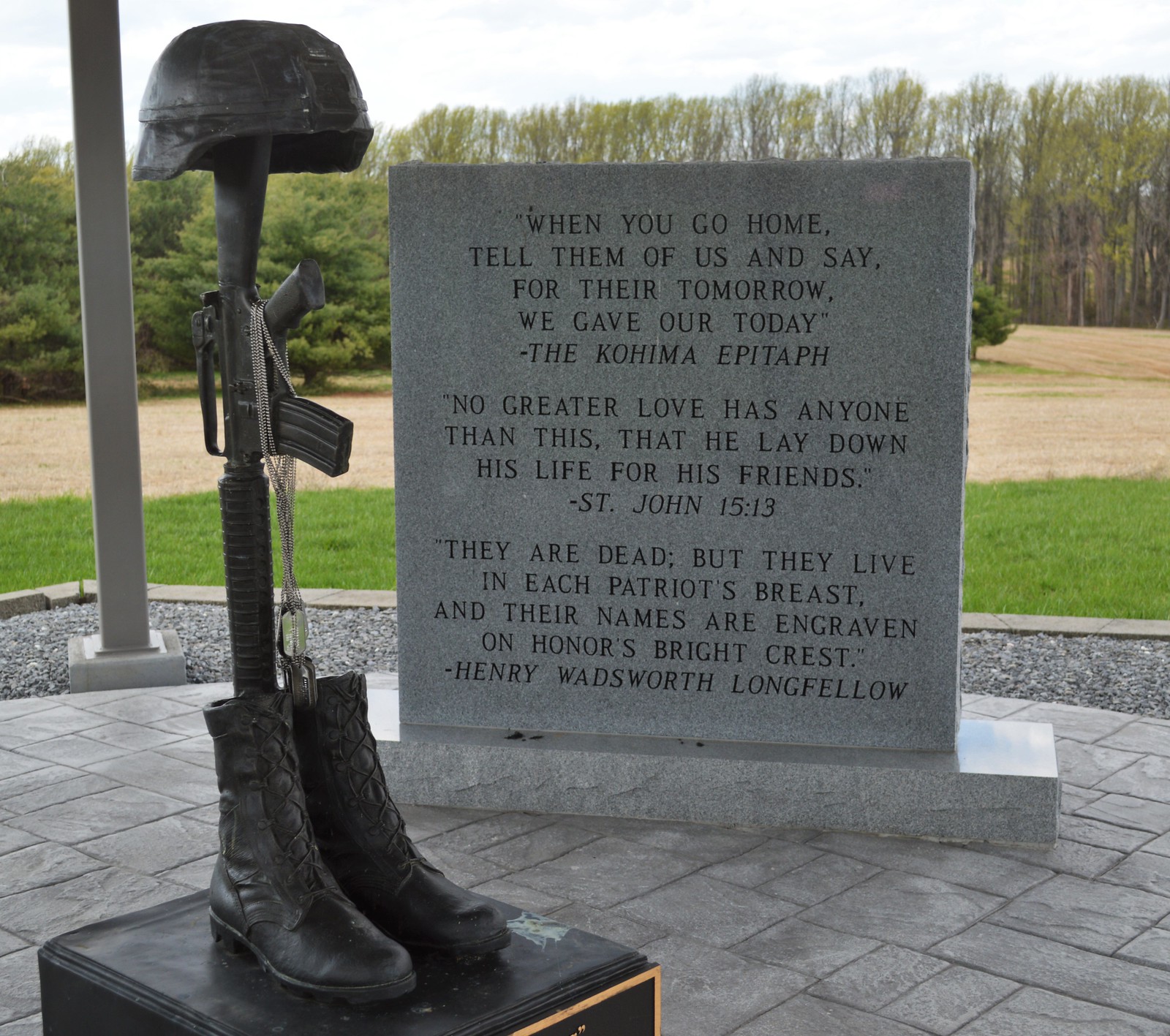This photograph captures an outdoor memorial dedicated to fallen soldiers, set against a serene backdrop of a field, a post, and a stand of green trees. The memorial consists of a prominent headstone inscribed with several poignant quotes: "When you go home, tell them of us and say, for their tomorrow, we gave our today," attributed to the Kohima Epitaph; "No greater love has anyone than this, that he lay down his life for his friends," from St. John 15:13; and "They are dead, but they live in each patriot's breast, and their names are engraven on honor's bright crest," by Henry Wadsworth Longfellow. In front of the headstone stands a powerful bronze sculpture, featuring a pair of combat boots with a rifle (likely an M16) propped up between them. Dog tags dangle from the rifle’s grip, and a helmet rests solemnly on its butt. The memorial evokes a strong sense of reverence and remembrance for those who sacrificed their lives for their country.